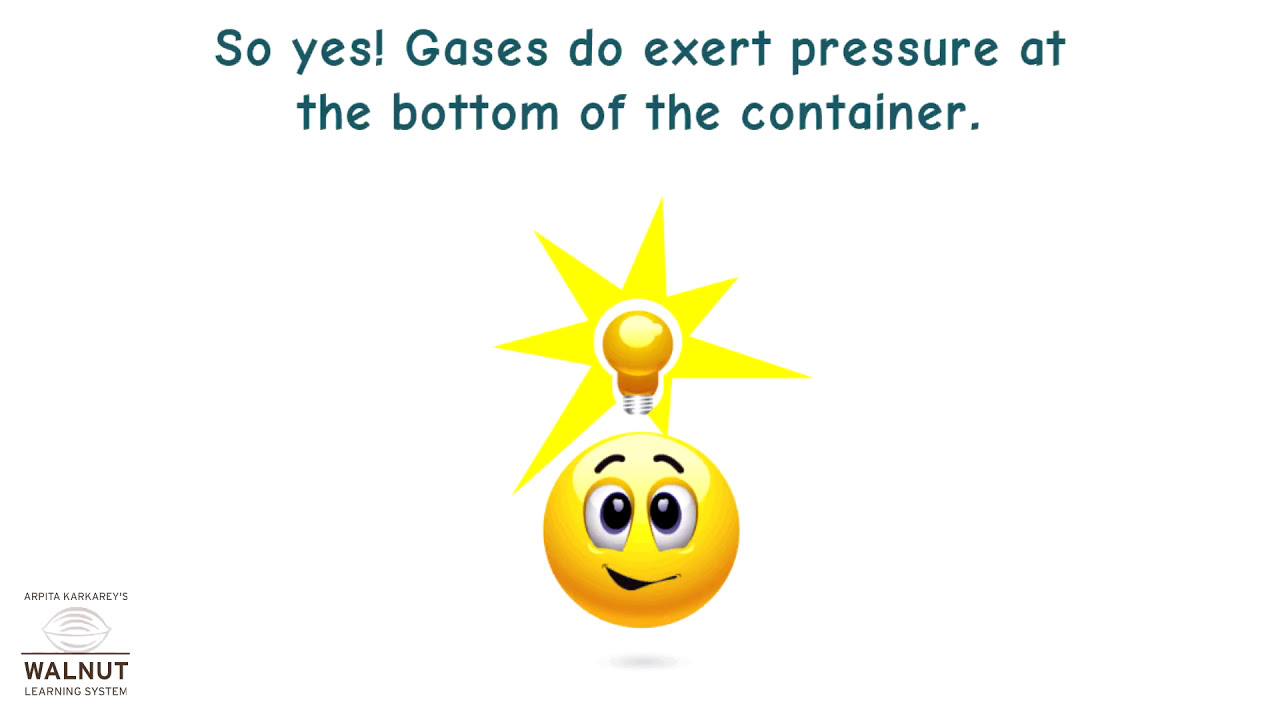The image appears to be a graphical element from an educational video. It features a white background with two lines of centered black text at the top reading, "So yes! Gases do exert pressure at the bottom of the container." Below this text is a 3D-rendered yellow emoji with a perplexed expression, including large, crossed eyes, and a slanted grin. The emoji has black eyebrows and a mouth. Positioned above the emoji's head is a lit yellow light bulb with a silver base, surrounded by a yellow action star, symbolizing a sudden idea. In the lower left-hand corner of the image is the logo and text “Arpita Karkariz” with an illustration of a walnut next to the text “Walnut Learning System.” The text "Walnut" is in bold, capitalized black letters, and the walnut illustration appears as a simple outline.